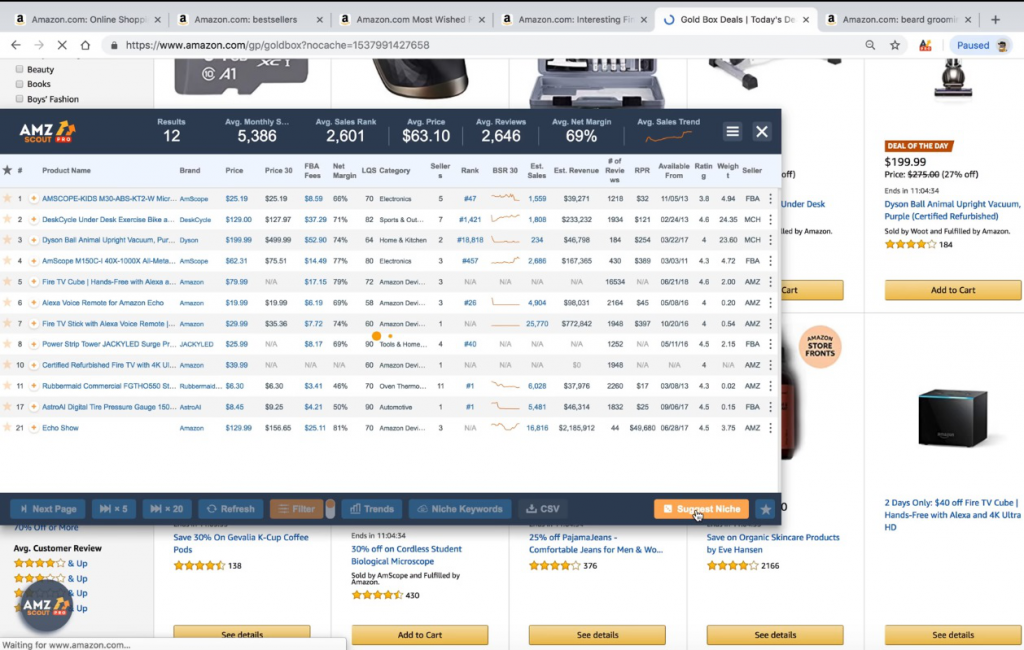This image displays an Amazon webpage with an overlay screen at its center. The top section of the Amazon site features a grey navigation bar with text that reads: "Amazon.com, online shop" followed by partially visible labels like "Amazon.com, best sellers," "Amazon.com, most wished," "Amazon.com, interesting" (which is cut off), "Gold Box Deals," and "Today's Deals," (abbreviated to "DE" and cut off), and lastly "Amazon.com, beard" (abridged and cut off).

Below this navigation bar are thumbnail images of products, complete with their prices and "Add to Cart" buttons. Superimposed upon this is a distinctive white box outlined in blue at the top and bottom. This box prominently houses "AMZScout" branding—where "AMZ" is in white—situated at the top. The topmost section of this overlay provides aggregate information with metrics that read: "Results: 12," "Average Monthly Sales: 5,386," "Average Sales Rank: 2,601," "Average Price: $63.10," "Average Reviews: 2,646," "Average Net Margin: 69%," and includes an "Average Sales Trend" accompanied by a small graph.

Below these summary statistics, the overlay displays detailed listings of items. Each listing includes the product's price, category, and rankings to offer an in-depth snapshot of market data on the platform.